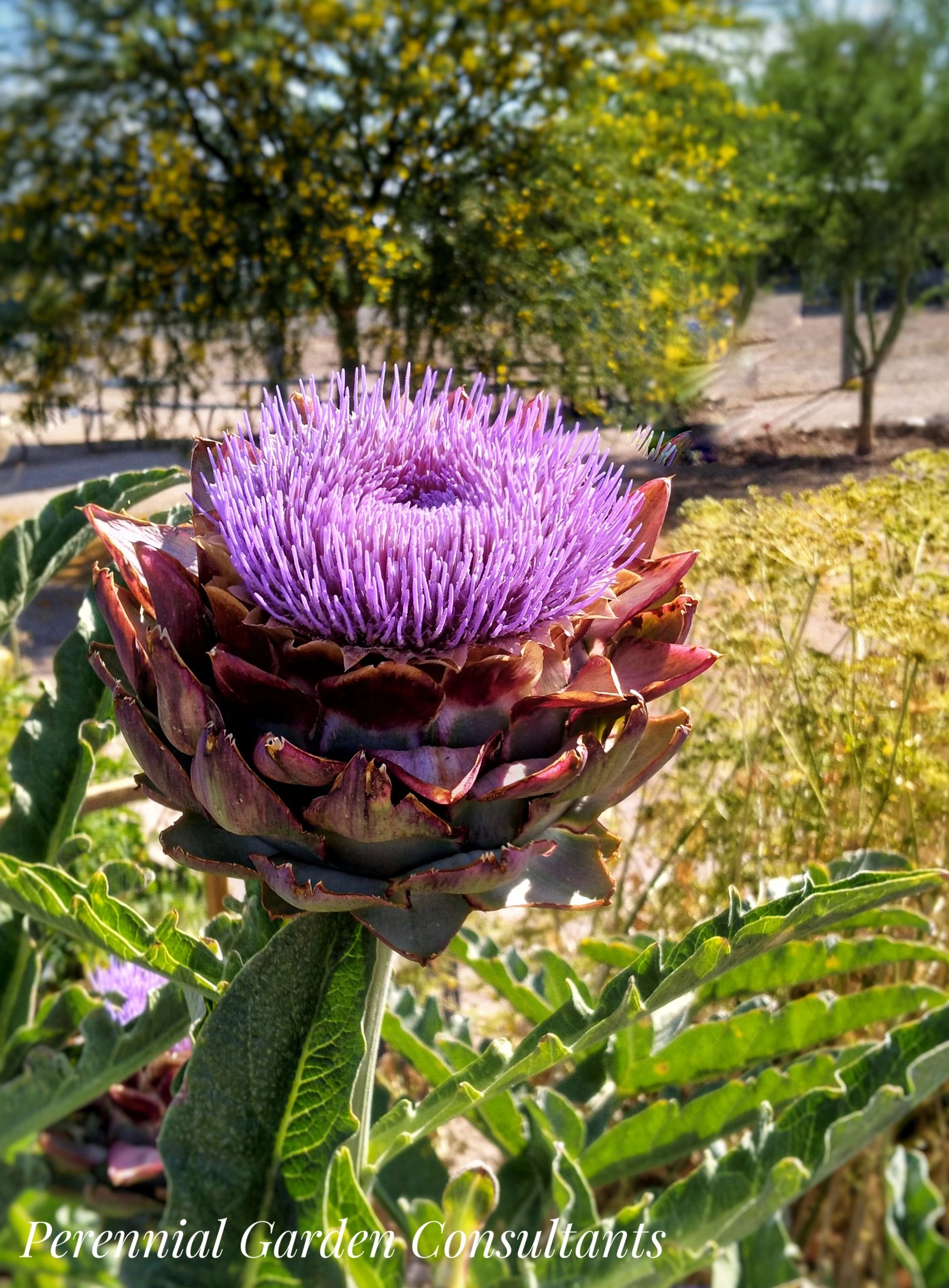This up-close photograph, taken by Perennial Garden Consultants as indicated by the white italic text at the bottom left-hand corner, captures the striking image of an artichoke that has fully opened and gone to bloom, nestled among fields of vibrant yarrow. The artichoke's leaves have spread wide, forming a bowl-like structure with spiky tips that have turned brown. Emerging from the center is a captivating purple flower, reminiscent of both an oceanic anemone and a zinnia, characterized by numerous purple spikes. Surrounding the main bloom are the spiky green leaves of the artichoke plant, and to its right, clusters of yellow yarrow flowers add a contrasting hue. In the background, a tree with some yellowing leaves stands against a bright, sunny sky, alongside some blurred greenery and possibly a walkway or water feature. The scene is devoid of any fauna or humans, focusing entirely on the beautiful interplay of the artichoke flower and the surrounding natural elements.